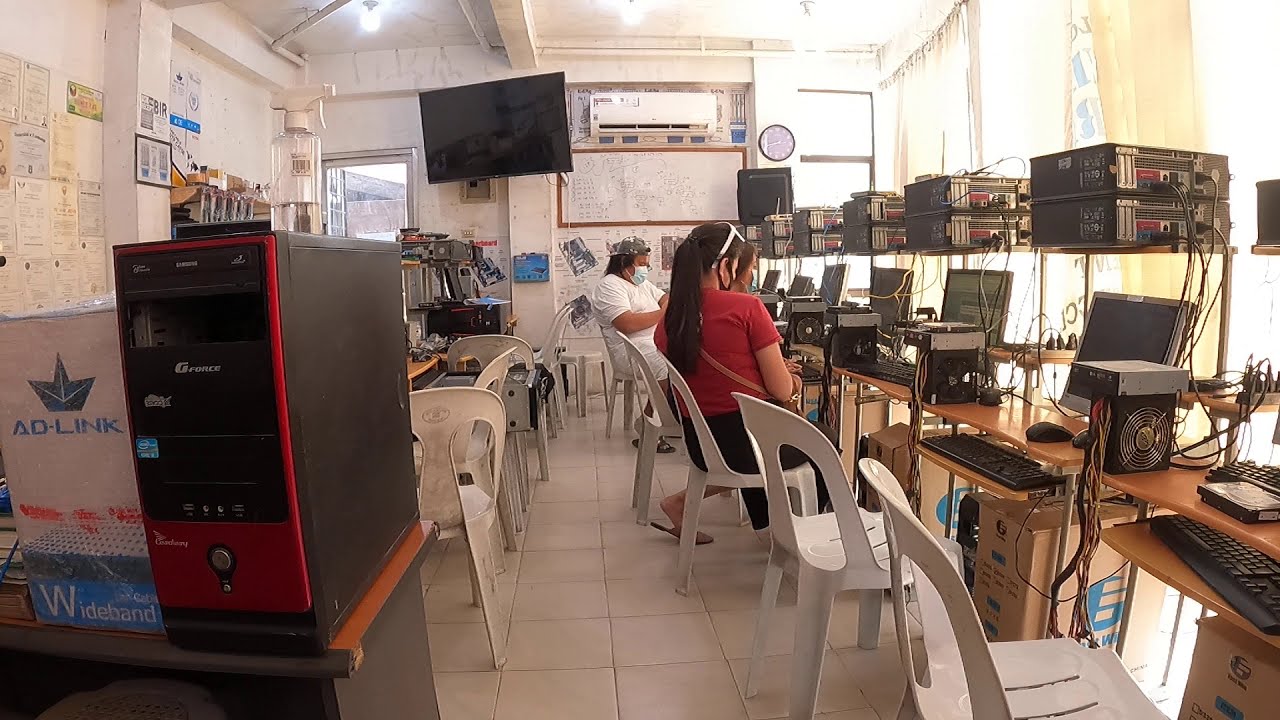In this detailed scene of an internet cafe, a small room is filled with numerous computer terminals, each equipped with a monitor, keyboard, CPU, and numerous connecting wires visible. White plastic chairs are placed in front of each terminal. The room has white tiled floors and walls, with windows adorned with thin curtains letting in ample light. Papers and cardboard boxes are scattered throughout, providing a glimpse into the utilitarian and slightly disordered environment.

To the left, there's a large wall-mounted TV screen while a whiteboard and various papers are pinned to the walls. In the background, a woman with long black hair in a ponytail, wearing a red T-shirt and black pants, is seated at a terminal. She has white sunglasses perched atop her head and appears to be carrying a crossbody bag. A man sits further back, donned in a white T-shirt, a baseball cap, and a face mask, emphasizing safety measures. This scene is representative of a developing country, possibly in Thailand or the Philippines. The networked setup of computers, with prominent black cable boxes above each terminal, suggests an activity possibly related to crypto mining or a similar intensive computer task.